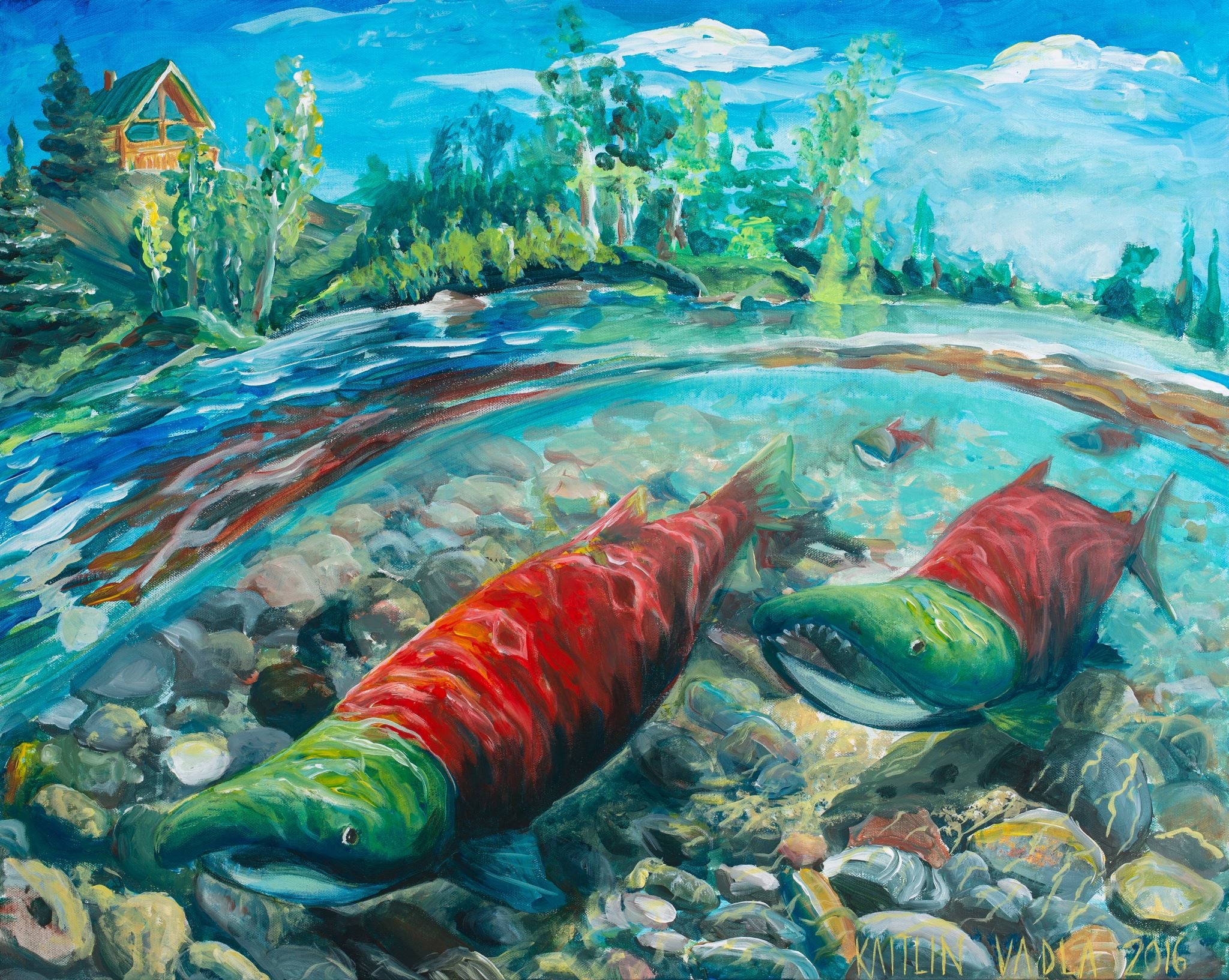This detailed oil-on-canvas painting by Caitlyn Vadla, dated 2016, showcases a serene natural scene. The horizontal, rectangular artwork primarily features a body of clear blue water—likely a river—in the foreground, populated with vibrant fish. The fish are distinctive with their green heads, long red bodies, and slightly green tails. Their sharp teeth add a unique character to them. Beneath the water, an array of rocks and stones is clearly visible, adding depth to the scene. The background presents a rustic log cabin nestled amongst numerous trees. The sky above is a rich blue with soft clouds, contributing to the painting's tranquil atmosphere. The artist's signature is found in the bottom right corner, ensuring the painting's authenticity and origin.